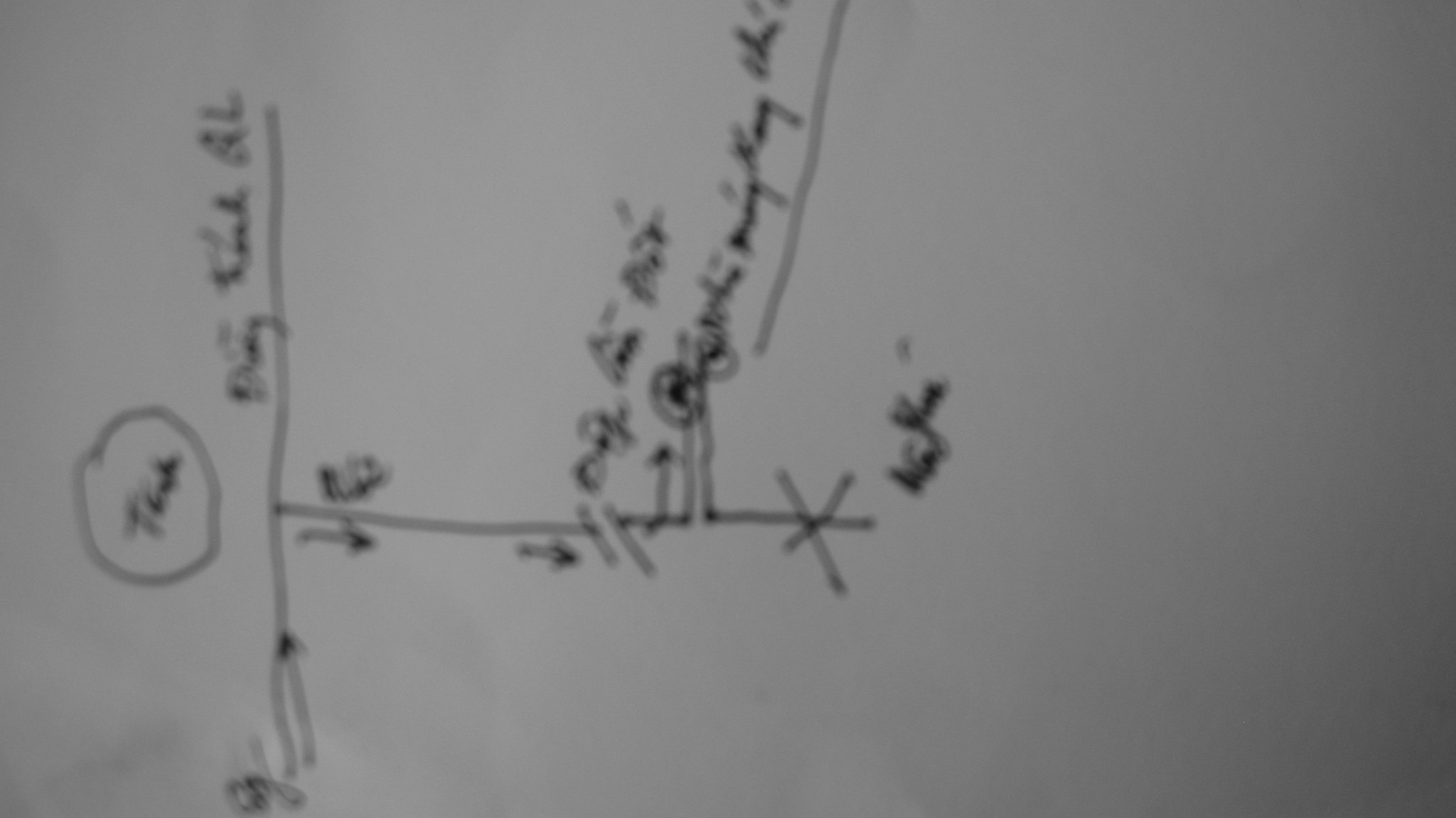The image depicts a blurred sketch on a white sheet of paper. The central figure in the sketch resembles a 'T' rotated 90 degrees counterclockwise. At the top of the horizontal line (now the vertical line due to the rotation), there is a circle containing some illegible words. Towards the right end of the same horizontal line, additional text is visible, though it's not clear enough to read.

The vertical line of the 'T' (now horizontal after rotation) features multiple arrows pointing downwards. Scattered across the lines are several 'X' marks and arrows branching out from the main lines. Additionally, two sets of parallel lines intersect the main horizontal line. These elements are accompanied by more text, which is also difficult to decipher, providing annotations or explanations. The overall impression is of a detailed and annotated diagram, though the blur obscures specific details and text.